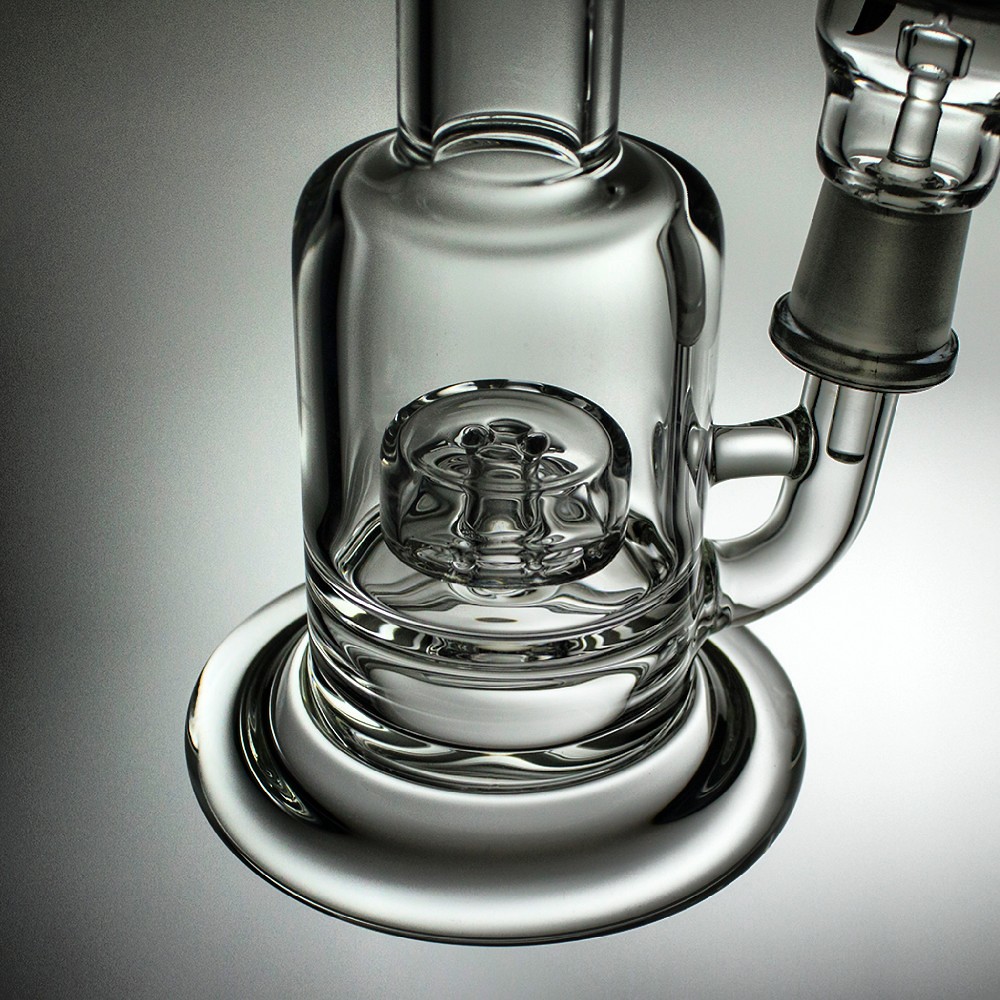The image features an intricately crafted, high-quality glass bong, showcasing detailed artistry and precision molding. Central to the composition is the transparent glass structure, within which lies a smaller, ashtray-like vaporizing piece encased in glass, surrounded by interconnecting tubes. The right section displays a sculpted piece extending upwards from the bong, culminating in a pipe and a smoke holder. The main body of the bong, partially extending beyond the image frame, reveals a flared base resembling a dish and a pedestal at the bottom. The entire device, though made of clear glass, exhibits variations in color, ranging from black to white and gray, emphasizing its clean and pristine condition. Set against a gradient background that transitions from light gray behind the bong to a darker edge, the overall presentation highlights the craftsmanship and elegance of this unique glassware.